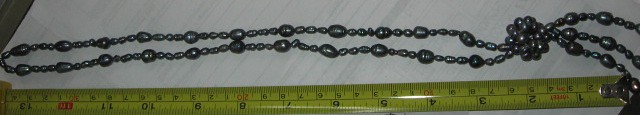The image is a detailed close-up of a beaded necklace laid on a white background that resembles a large sheet of lined paper. The necklace consists of small, dark gray beads interspersed with larger beads, following a recurring pattern. Towards the right side, there's a knot from which the necklace branches into three separate strands. The necklace is aligned with a yellow measuring tape that spans from 1 to 13 inches, helping illustrate its significant length. The measuring tape features black numbers and red markings for specific measurements. Also visible in the upper left corner is a dark wooden surface, suggesting the white background is placed on another surface. Near the top, there's a cluster resembling a bundle of beads, adding to the intricate design of the necklace. The overall scene provides a clear view of the necklace's structure and length, juxtaposed against the precisely marked measuring tape.